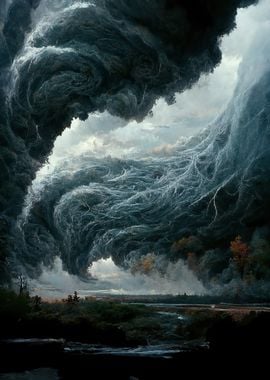The painting depicts a dark and turbulent landscape dominated by a dramatic and abstract sky. The upper half of the image is filled with ominous, stringy clouds that stretch across the canvas, creating a haunting atmosphere. These clouds are an intricate blend of dark gray, black, and varying shades of blue, forming twisted, vein-like structures that resemble clusters of strings. One massive cloud formation looms in the upper left corner, while another stretches diagonally from the lower left to the upper right, with patches of clearer sky and white clouds interspersed, allowing glimpses of blue sky to peek through.

Below this chaotic sky, the lower portion of the painting is shrouded in darkness, but you can discern a landscape of trees, shrubs, and what appears to be a field on the right. A river or stream meanders through the scene, bordered by the silhouettes of trees and a few rocks in the foreground. Despite the eerie tone set by the tumultuous sky, the land and water below add a grounding element to the dramatic composition.